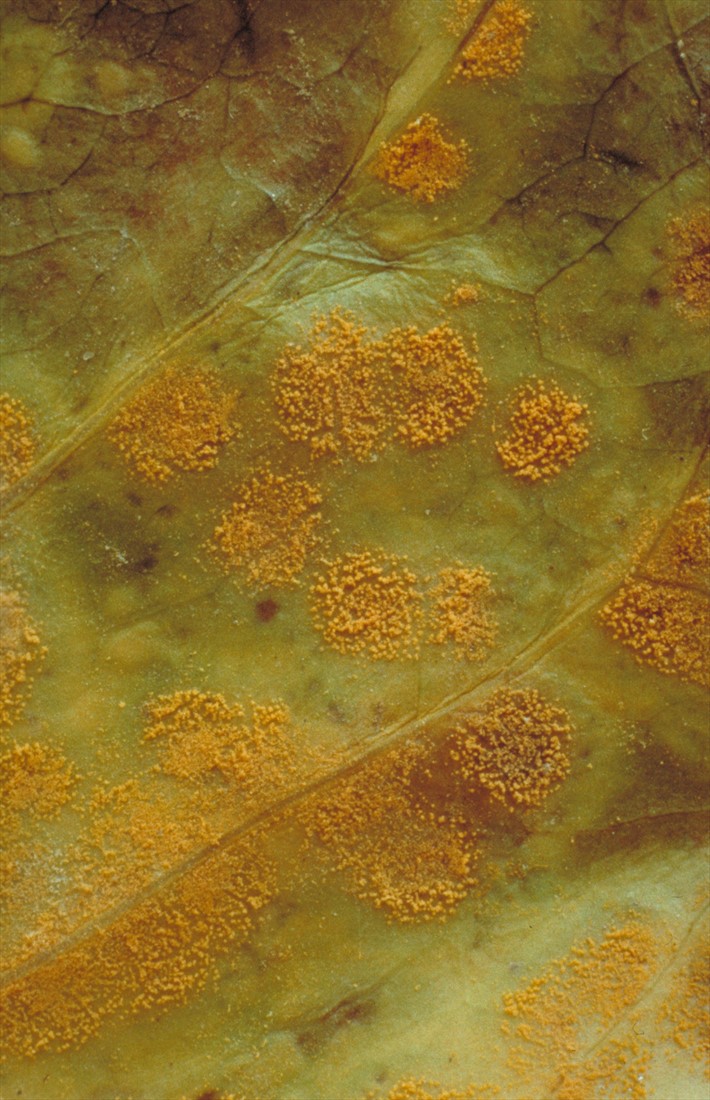The image is a highly detailed, close-up shot of a single leaf. The primary color is green, with the background featuring a lighter green hue. This leaf showcases a network of veins that vary in color, with most appearing black or dark brown, while a few retain a lighter green shade. Notably, some areas of the leaf have a sandy-like texture, presenting in a lighter brown color. This texture is especially prominent in the bottom right and central parts of the leaf, while the top left corner is devoid of this feature.

Scattered across the leaf are yellowish specks, resembling seasoned powder such as cinnamon. These specks are distributed from the top to the bottom of the image, adding to the complexity. Additionally, small black dots are interspersed among these specks, creating an even more intricate pattern. The overall surface of the leaf appears flat and soft, with its detailed veins and varied textures forming a rich tableau that could be observed under a microscope or a close-up lens, lending a microscopic feel to the image.